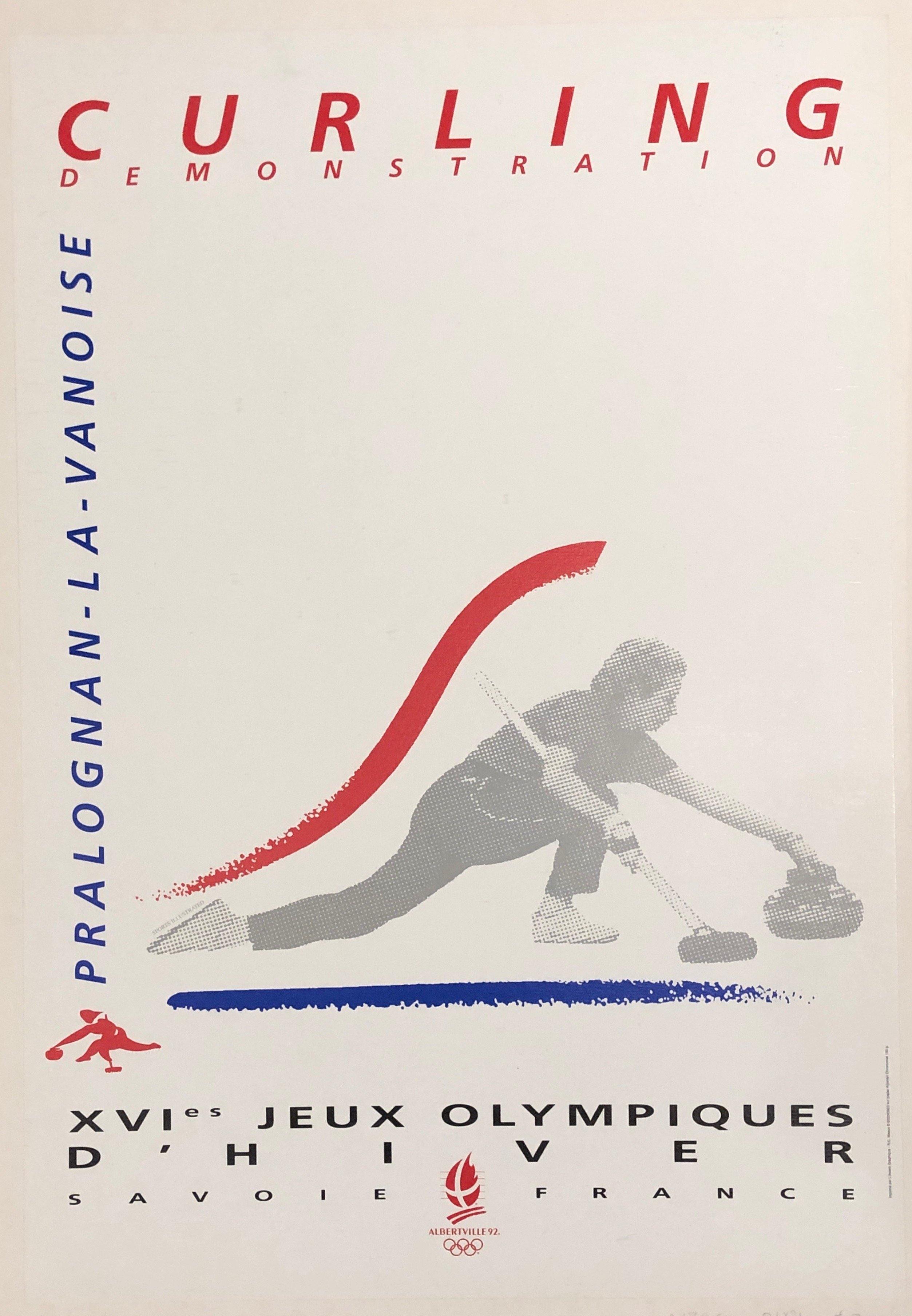**Curling Demonstration**

This captivating image, set on an off-white background, serves as a promotional flyer. At its heart is a dynamic, black and white, slightly pixelated portrayal of a woman in the midst of executing a curling throw. She leans forward, forming an elegant S-shape with her body, her right knee bent and her left leg extended behind her. Her left hand reaches out, gently guiding the curling rock, while her right hand grips a curling broom with precision.

Above her, a red line arcs upward, adding a sense of motion and energy to the scene. Below, a horizontal blue line stretches across, grounding the composition. 

On the left side of the flyer, text reads vertically from bottom to top: "Prelogin la Venice," accompanied by additional text in French. Beneath this, the iconic Olympic symbol is displayed with a red flame, marking the event as a part of the Albertville 1992 Winter Olympics.